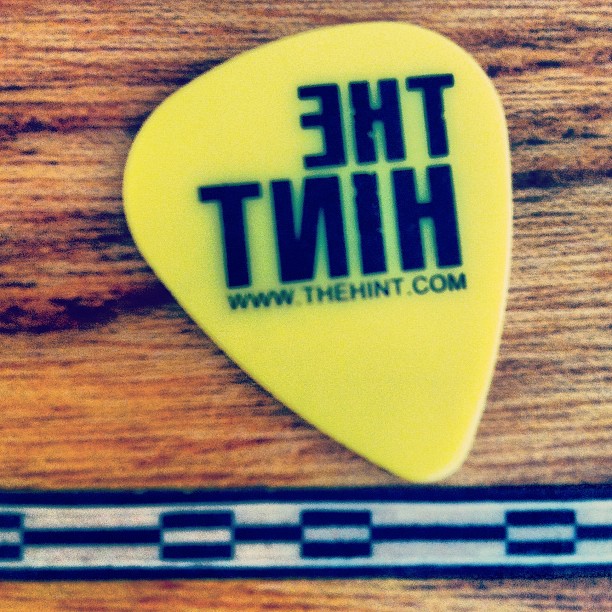The image is a zoomed-in view of a yellow guitar pick featuring the text "THE HINT" in capital letters, printed in blue and appearing reversed. Directly below, the web address "www.thehint.com," also in blue, is printed on the pick's surface. The guitar pick, which has a rounded shape with a slightly oval top, lies flat on a brown wooden surface displaying visible wood grains. At the bottom of the image, there's an abstract, repetitive blue and white striped pattern. The overall composition suggests the pick might be resting on a guitar or a wooden table.